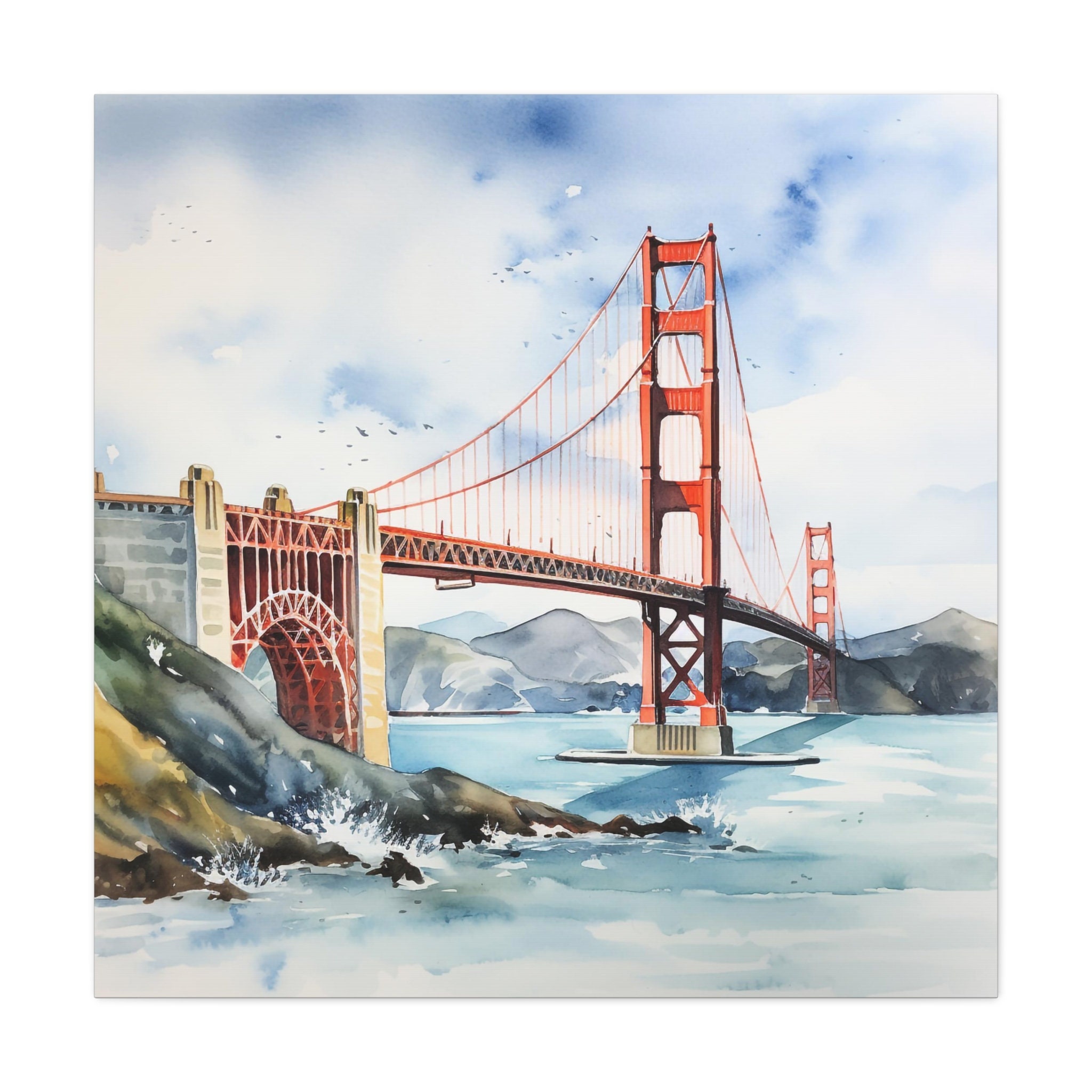This watercolor painting captures a vivid, full-color scene featuring the iconic Golden Gate Bridge from a perspective along one side, looking down its length. The bridge, characterized by its red towers, with two visible towers—one in the middle of the composition and one in the far distance—spans a large body of water. The colors used in the painting are predominantly pastels, with a palette featuring light greens, blues, browns, and greys. The bridge’s red contrasts sharply against a sky that is mostly occupied by wispy white clouds, with only faint hints of blue, making the structure stand out prominently. Below, the water is depicted in light, pale blue hues, with splashes of white foam where waves crash against the rocky, brown shore. In the background, opposite the bridge, there are dark brown and green mountains, adding depth and context to the serene, yet dynamic scene.